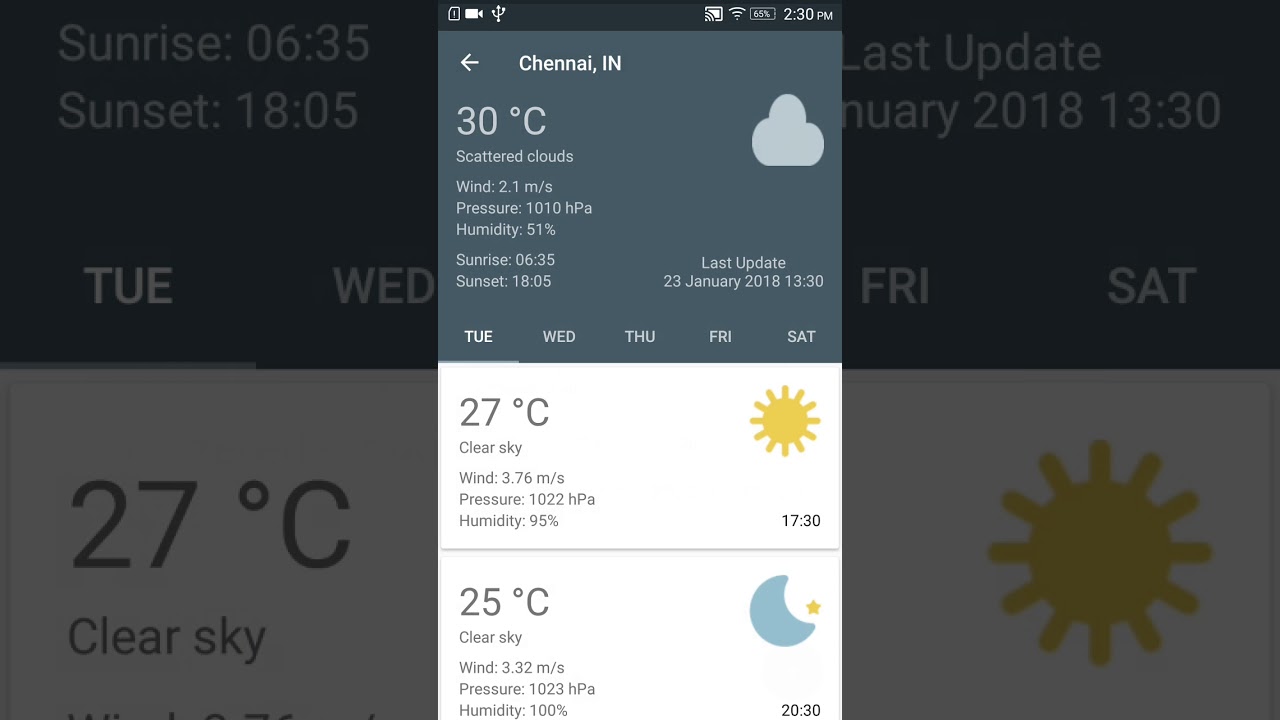**Detailed Caption:**

The screenshot displays a weather app interface on a smartphone. In the background, there is an enlarged, blurry version of the app with a gray overlay, emphasizing the actual weather information panel in the foreground. This central panel is narrow and runs vertically down the screen, resembling a typical phone display.

At the top of the screen, various icons are present: a video camera icon, a USB icon, a screen share option, a full Wi-Fi symbol, and a battery meter showing approximately 55%. The time is indicated as 2:30 PM. Below these icons, the background color shifts to a desaturated slate gray.

The weather information shows that the current location is Chennai, India, with a temperature of 30°C and scattered clouds. An icon of a cloud appears on the right. Additional weather details include a wind speed of 2.1 meters per second, atmospheric pressure of 1010 HPA, and humidity at 51%. Sunrise is at 6:35 AM, and sunset is at 6:05 PM. The last app update was on January 23rd, 2018, at 1:30 PM.

The app displays a five-day forecast with tabs for Tuesday, Wednesday, Thursday, Friday, and Saturday, with Tuesday currently selected. Below the weekday tabs, two weather snapshots are provided:

1. At 5:30 PM, the temperature is 27°C under a clear sky, depicted with a sun icon. The wind speed is 3.75 meters per second, pressure is 1022 HPA, and humidity is 95%.
   
2. At 8:30 PM, the temperature drops to 25°C, also under a clear sky, illustrated by a moon and star icon. The wind speed is 3.32 meters per second, pressure is 1023 HPA, and humidity is at 100%.